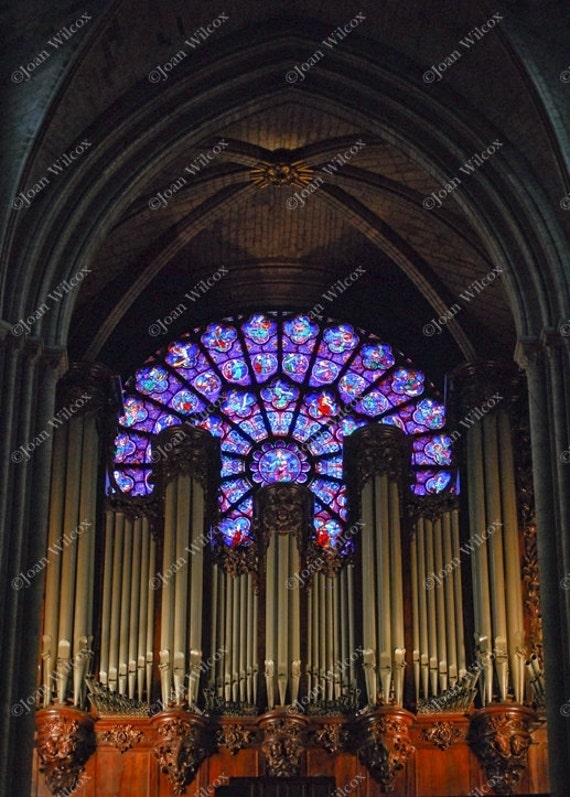The photograph captures the intricate interior of a medieval European cathedral, focusing on a grand, elaborate church organ. The top of the organ features large, well-polished, metallic pipes integrated into gothic architecture. Beneath the pipes, there is an intricately carved wooden structure, displaying dark red hues and eccentric designs, possibly adorned with visages or lion motifs. Above, the stone arch ceiling of the cathedral is visible, showcasing traditional European craftsmanship. Behind the organ, a magnificent circular stained-glass window dominates the scene with its sophisticated array of purple, blue, red, yellow, and white colors, forming swirling patterns. The entire image is overlaid with a transparent yet repetitive watermark reading “Joan Wilcox,” stamped diagonally across the photograph more than 30 times.